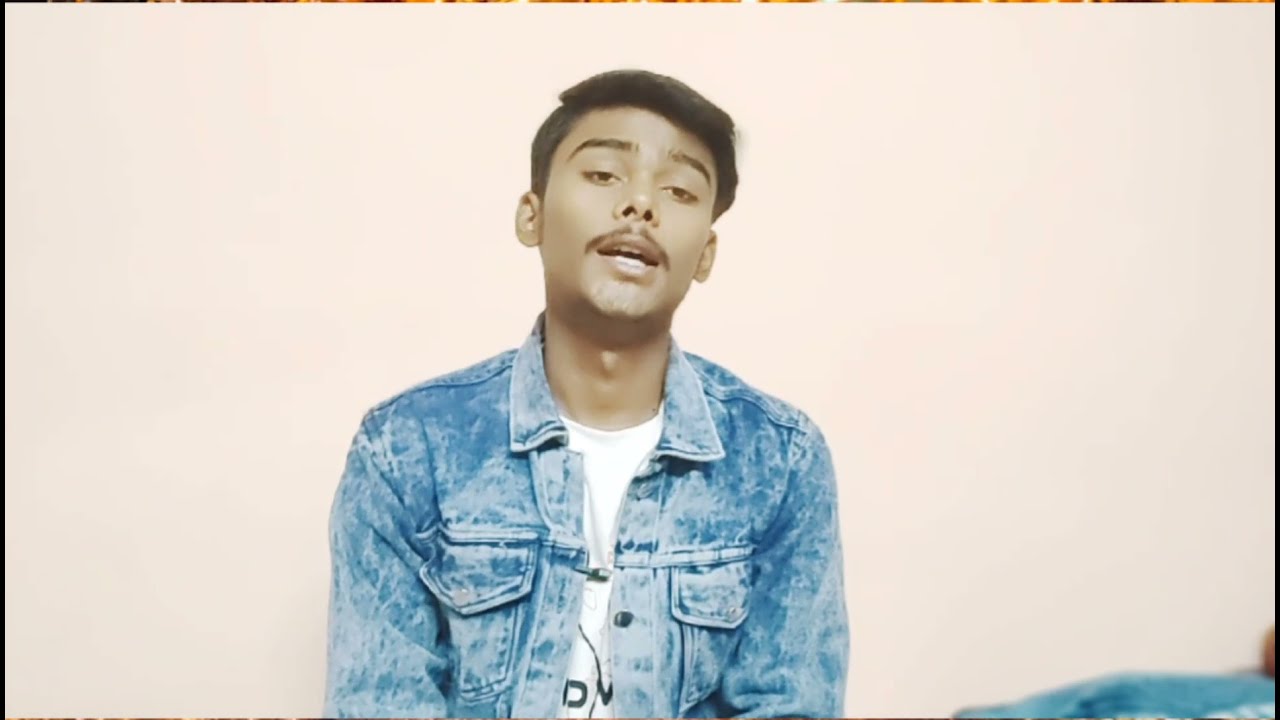This photograph features a young man, possibly in his 20s, seated indoors against a light pink wall. He's centrally positioned in the frame, sporting a casual yet confident demeanor with his mouth open, mid-speech. His complexion is tan or brown, potentially indicating Indian or Hispanic heritage. He has striking black hair, slightly closed brown eyes, and a thin mustache. He is dressed in a white t-shirt with partially visible letters "D.M." underneath an open blue jean jacket that has two front pockets. The overall vibe suggests he might be making a video, possibly sharing his thoughts or giving a talk. There are no other people in the room, although there appears to be a table with a blue tablecloth in the lower right corner of the image.